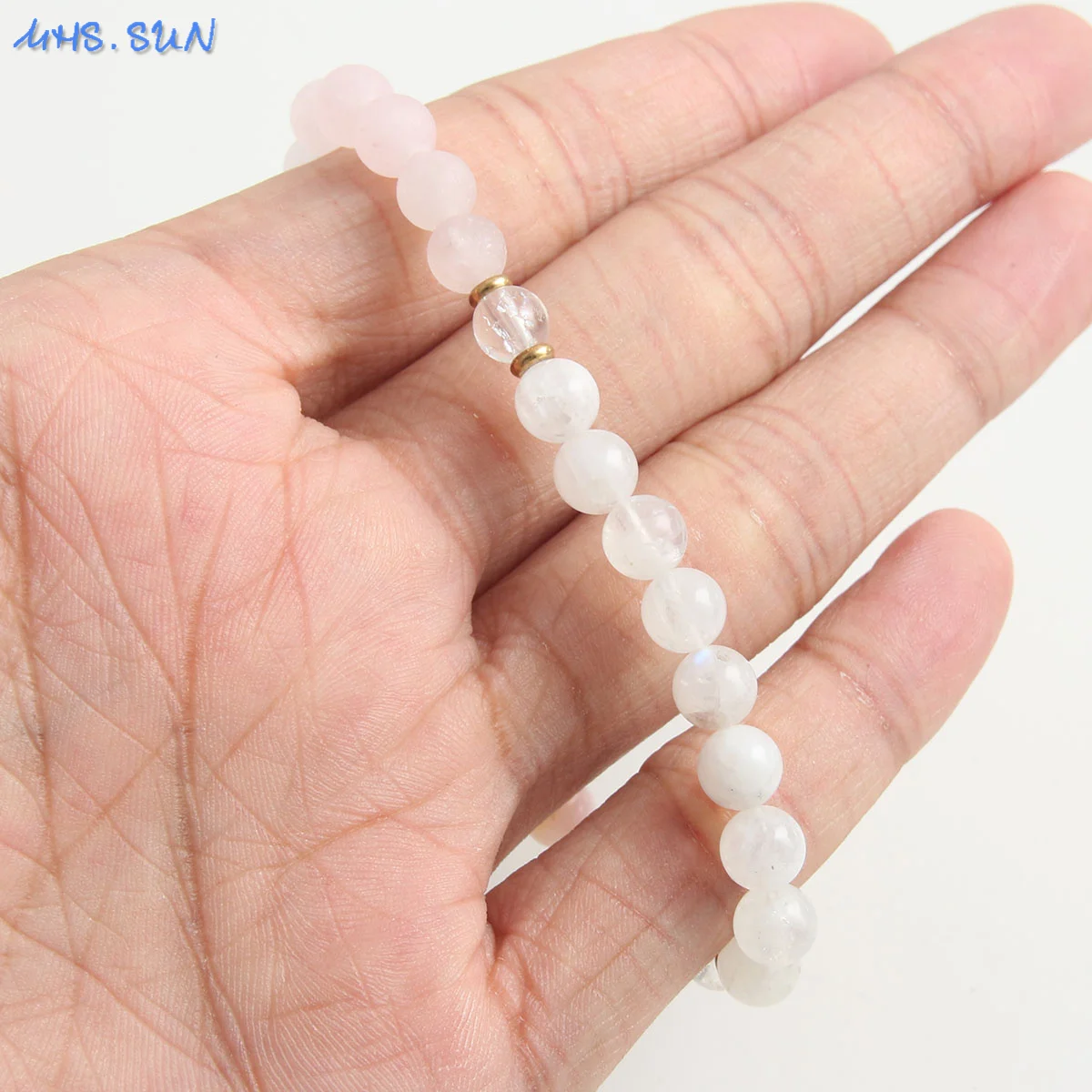The image features a close-up of a wrinkled Caucasian hand holding a delicate white bead bracelet through the fingers. The beads are primarily opaque white with a marble finish, except for a single transparent bead in the center, flanked by two tiny gold clasps. The person is showcasing the bracelet against a stark white background, possibly for advertisement purposes. In the top left corner, the only text appears in blue cursive, reading "mhs.sun," with the background slightly darker in that area.